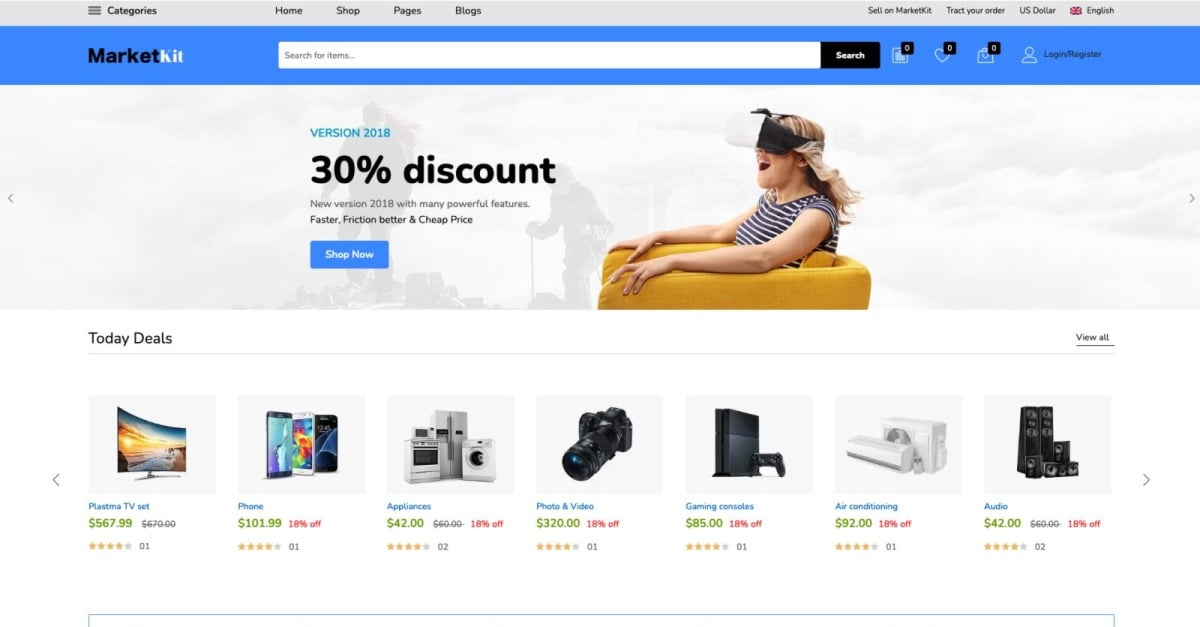In this detailed image of an e-commerce website interface, prominently titled "Market Kit", a sophisticated online shopping platform is showcased. The website's name is displayed in the top left corner, with the word "Market" rendered in black and "Kit" in white for a striking visual contrast. Adjacent to the name, there's a functional search bar designed for user convenience; it invites users to "search for items" on the far left, and features a black "Search" button on the far right.

To the right of the search bar are three navigational icons, each symbolizing a different function: a square icon, a heart icon for favoriting items, and a camera icon. Additionally, there is a profile icon prompting users to "Login" or "Register" for a personalized experience.

Dominating the center of the image is a lively picture of a woman with a white skin tone. She sits comfortably in a chair, donning a VR headset and displaying an expression of elation. The woman features blonde hair and is dressed in a black shirt with white stripes, adding to the contemporary feel of the scene.

To the left of this dynamic image, promotional text draws attention to a "Verizon 2018 30% discount." It highlights the "New version 2018" of a product, touting its "many powerful features," including increased speed, better friction, and an attractive price point. Below this enticing advertisement is a call-to-action button urging viewers to "Shop Now."

At the very bottom of the image, an assortment of product thumbnails is showcased in a horizontal lineup. These products include, from left to right: a television, a smartphone, kitchen appliances such as a refrigerator, oven, and dryer, as well as a camera, a PlayStation 4 gaming console, an air conditioner, and an audio product. Each thumbnail invites potential shoppers to explore the diverse range of items available on Market Kit.